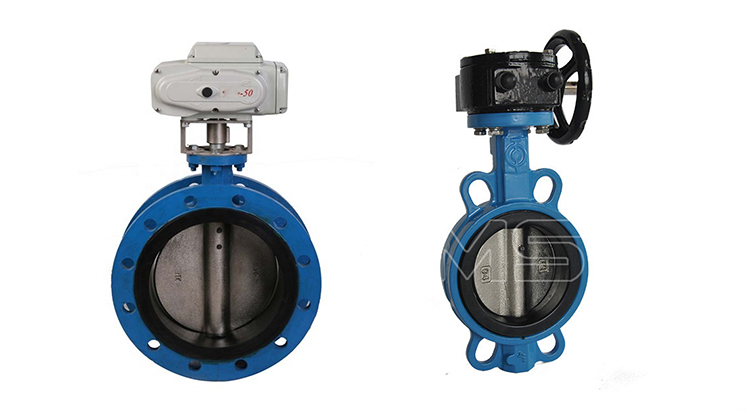The image depicts two large water shutoff valves standing upright, each with a predominantly blue circular housing. Both valves are designed with an inner mechanism to regulate fluid flow via a metal gate that flaps open and closed. The valve on the left features a white or gray top box, engraved with the number "50" in red, and the center includes a black ring and silver component with round bolt holes surrounding the perimeter. This valve appears to be electronically operated, given its lack of a manual control wheel. The valve on the right has a black upper section with a hand-operated black gear wheel for manual operation. An identifiable silver bar is visible, extending either through or behind the wheel, with the center section including a black and gray combination. The housing for both valves is adorned with metal accents, and the entire setup is set against a white background.